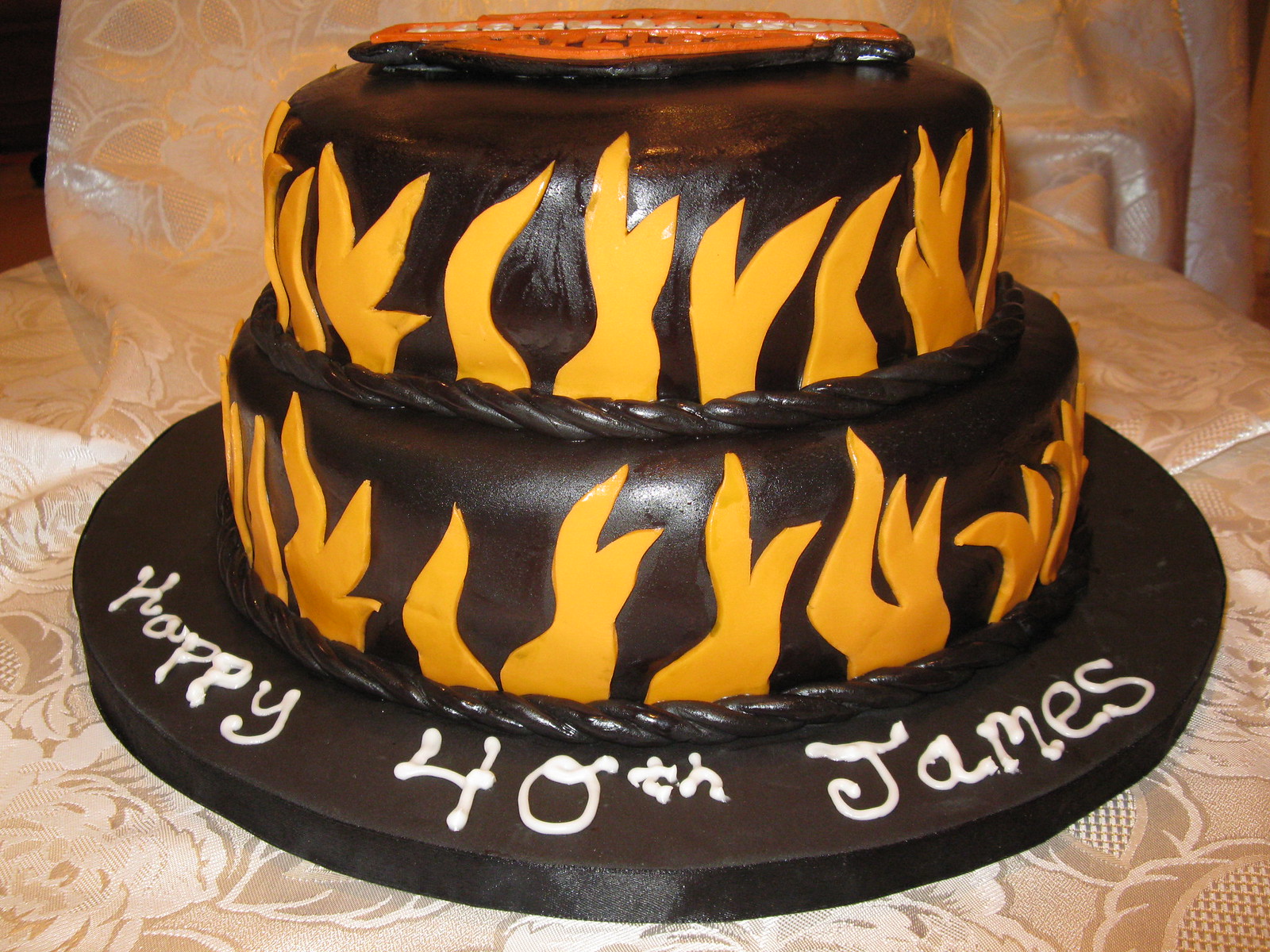In the center of a light whitish peach tablecloth featuring a subtle floral pattern, there is a striking birthday cake. The cake consists of two layers, each adorned with orange and yellow flames that rise vertically from the base. The bottom layer is round and styled to resemble a tire, while the smaller second layer mimics the same design. The entire cake is set on a black base, where the message "Happy 40th James" is written in white icing. The topmost layer displays an orange and beige emblem, possibly a Harley-Davidson logo, though it is partially obscured by the angle of the photograph. This detailed and unique cake, captured in an amateur photograph likely shared on social media, celebrates James' milestone birthday with its bold colors and intricate design.